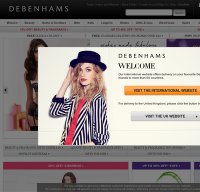In this image, there is a small, slightly blurred screenshot of a Debenhams webpage. Prominently displayed is a pop-out dialog box with a welcome message from Debenhams. The text within the dialog is mostly unreadable due to the fuzziness, but it's clear that there is an orange button with unreadable text likely indicating an action to be taken, such as 'Shop Now' or 'Learn More.' Below the orange button, there’s a gray button with unreadable text and a small black arrow pointing to the right, possibly indicating further navigation or options pertaining to the website.

On the left side of the dialog box, there's a photograph of a woman with long blonde hair wearing a hat. She is holding a blue hat with her right arm placed on top of her head. The woman is dressed in a blue and white striped blouse or jacket, featuring three-quarter length sleeves, and underneath, she is wearing a red shirt or possibly a red tie.

Behind the dialog box, the Debenhams webpage is faintly visible, showing a menu bar at the top, likely containing various shopping categories or navigation links. The overall scene suggests a promotional or welcome message for visitors landing on the Debenhams site, aiming to guide them through specific actions or offers.